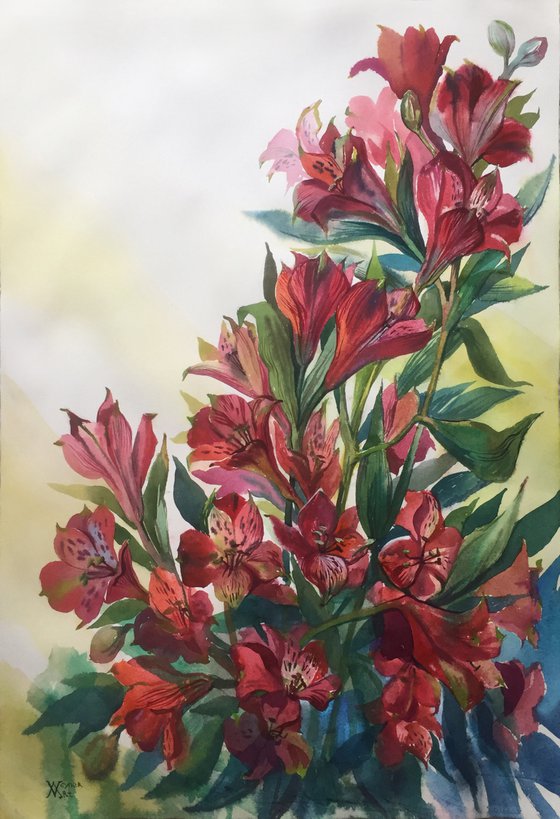This is a vibrant watercolor painting depicting tall red lilies at various stages of bloom, with some flowers fully open while others remain tight buds poised to blossom. The lilies are accentuated by lush, dark green leaves, some of which face directly towards the viewer while others are viewed from the side, showcasing the flowers' detailed insides and delicate petals. The realistic composition features subtle blue hues near the bottom and a backdrop that transitions from blurred white to yellow, suggesting a softly lit outdoor setting. Darker specks and shading within the petals add depth and texture, while long, yellow tendrils extend from the flowers. A signature marked with a large "W" and "M" in black font is present in the far left corner, grounding the piece.